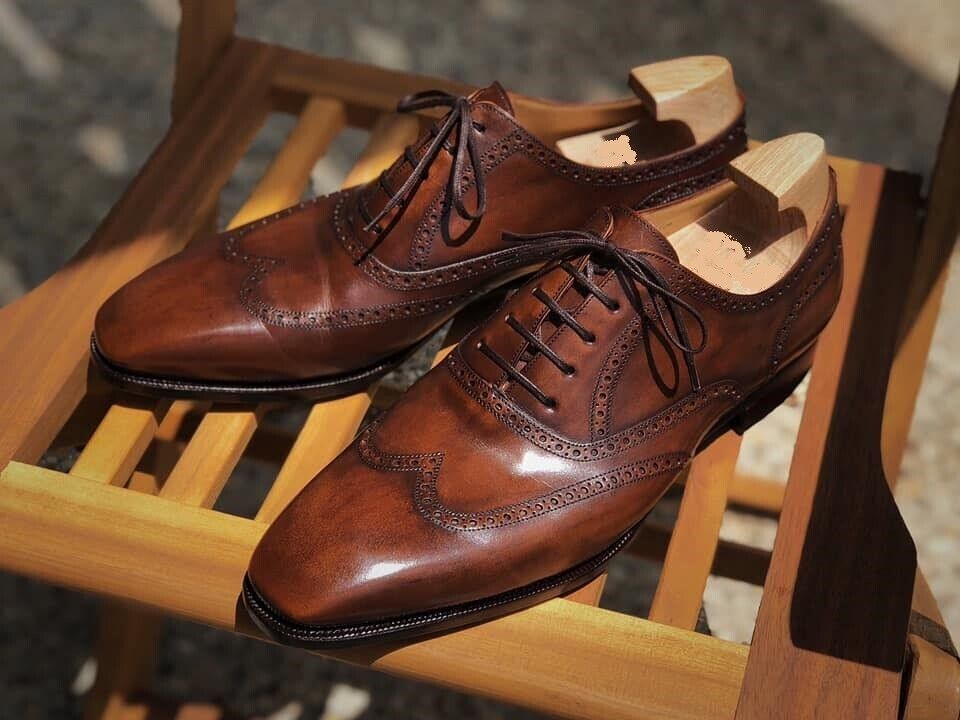This image features a pair of medium brown leather oxford dress shoes with dark brown laces, sitting on a medium brown wooden chair with an open back and eight slats. The shoes each contain wooden shoe trees, designed to maintain the shoes' shape over time. The shoe trees have small handles or knobs to facilitate easy removal. The shoes boast intricate stitching details that extend from the pointed toes up to the laces and around the sides, ending just above the black soles. The setting is a light gray, brownish surface, further accentuating the elegant and well-kept appearance of the shoes.